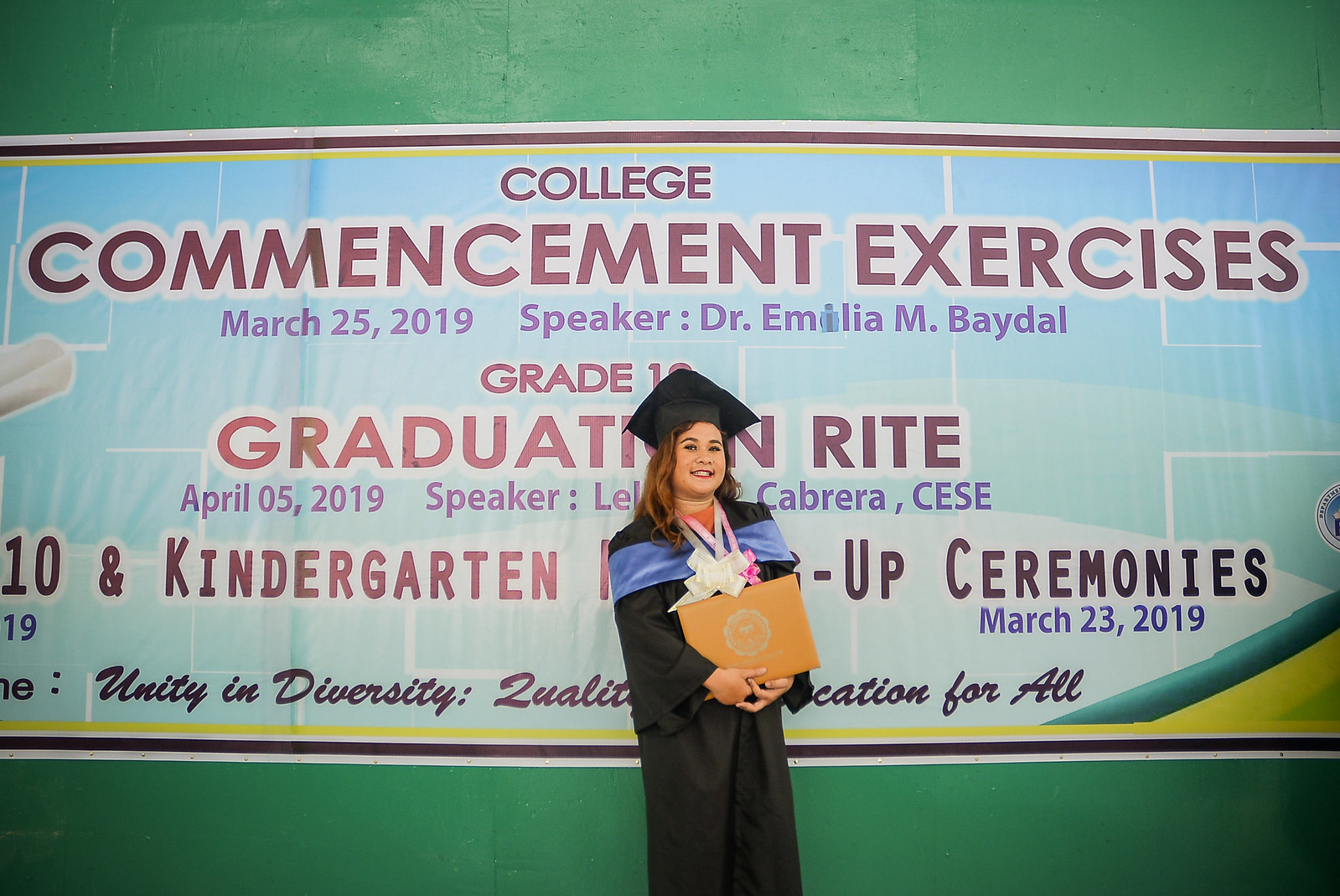The image is a landscape-oriented color photograph of a young woman with light brown skin, standing against a backdrop featuring a detailed banner. She is at a graduation ceremony, donned in full regalia, which includes a black graduation cap and gown, along with pink and purple lanyards draped across her chest. She is holding a blue diploma in her hands.

The background banner behind her is dominantly light blue with vibrant text in red, blue, and yellow, framed by white drop shadow. At the top, the banner announces "College Commencement Exercises." Below this, it provides the date "March 25th, 2019" and mentions the speaker, "Dr. Amelia M. Badall." Further down, amidst more dates and event details partially obscured by the graduate's cap, the text includes phrases like "grade graduation" and references to other ceremonies on "April 05, 2019" featuring a speaker with the last name "Cabrera," and additional kindergarten ceremonies dated "March 23rd, 2019." The catchphrase "University in Diversity" is positioned at the bottom of the banner.

The green paint spanning the top and bottom sections of the wall complements the blue background of the banner, bringing a cohesive color palette to the scene. The overall aesthetic and intricate details within the photograph align with the style of photographic representational realism.